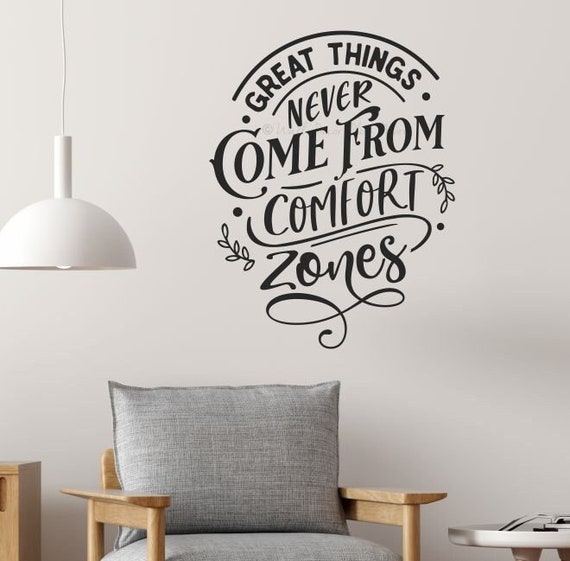The image depicts a serene room with a white wall serving as the backdrop. Centrally positioned in the frame is a wooden chair adorned with grayish, almost silver pillows on both the backrest and the seat. To the chair’s left, a substantial white lamp with a half-circle head hangs from the ceiling by a slender, white wire. On the right side of the chair, partially visible, stands a white table supported by wooden slats, on which rests a pair of glasses and some books. Just above the chair on the wall, an inspirational quote is artistically displayed in varied black lettering, stating, "Great things never come from comfort zones." The overall composition blends elements of comfort and motivation within a modest yet aesthetic setting.